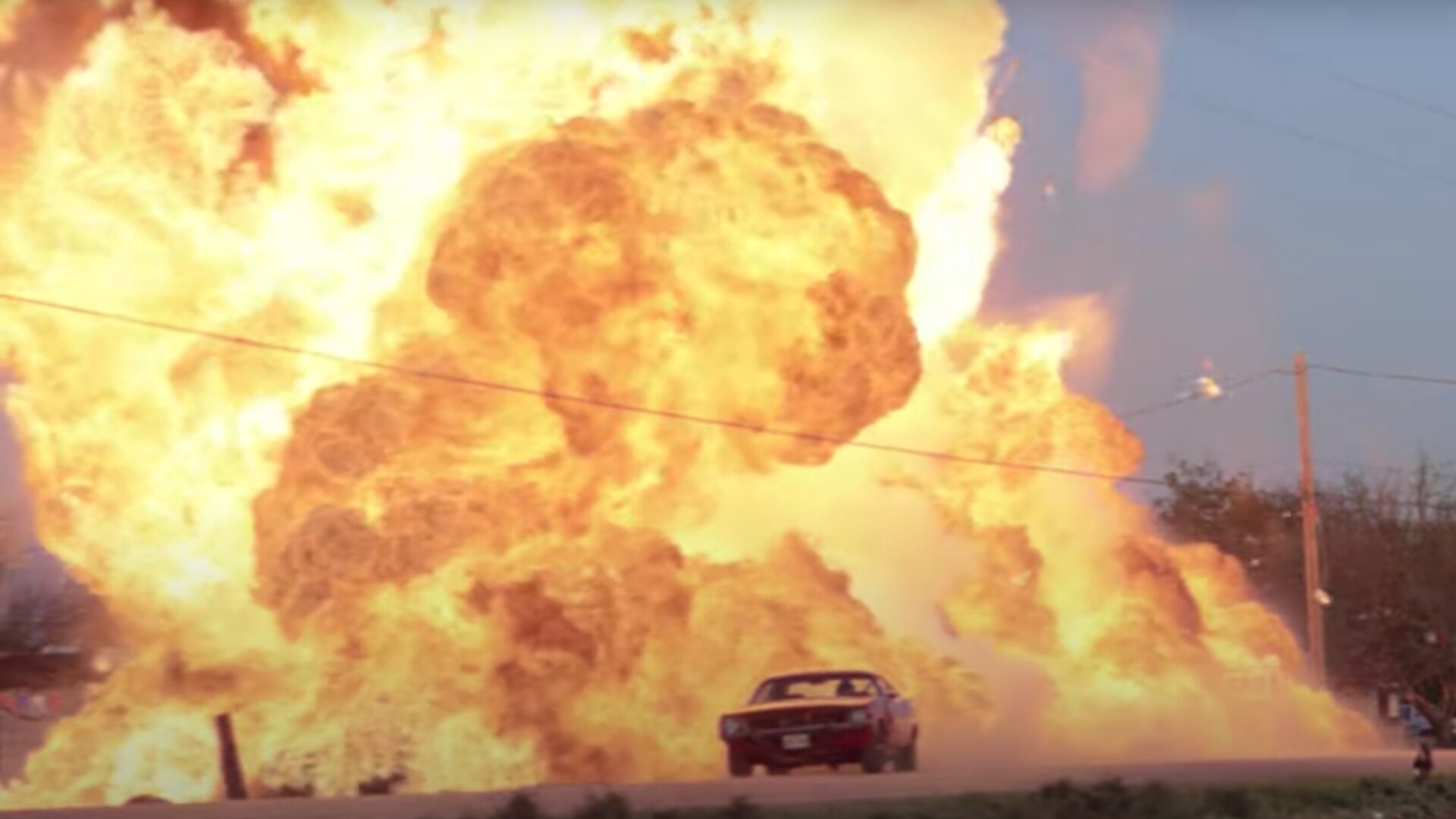A vintage, reddish 1970s-style vehicle speeds away from a massive explosion, leaving behind a roaring fireball of black, yellow, and orange hues. The scene is framed by a scattering of power lines, both in front of and behind the car, and a prominent wooden post. Lush green trees create a backdrop, while the road stretches out beneath a partly visible sky. The foreground features patches of green grass in varying shades, adding depth and contrast to the image. The photograph, slightly grainy but excellently preserved, captures the dynamic intensity of the moment with remarkable clarity.